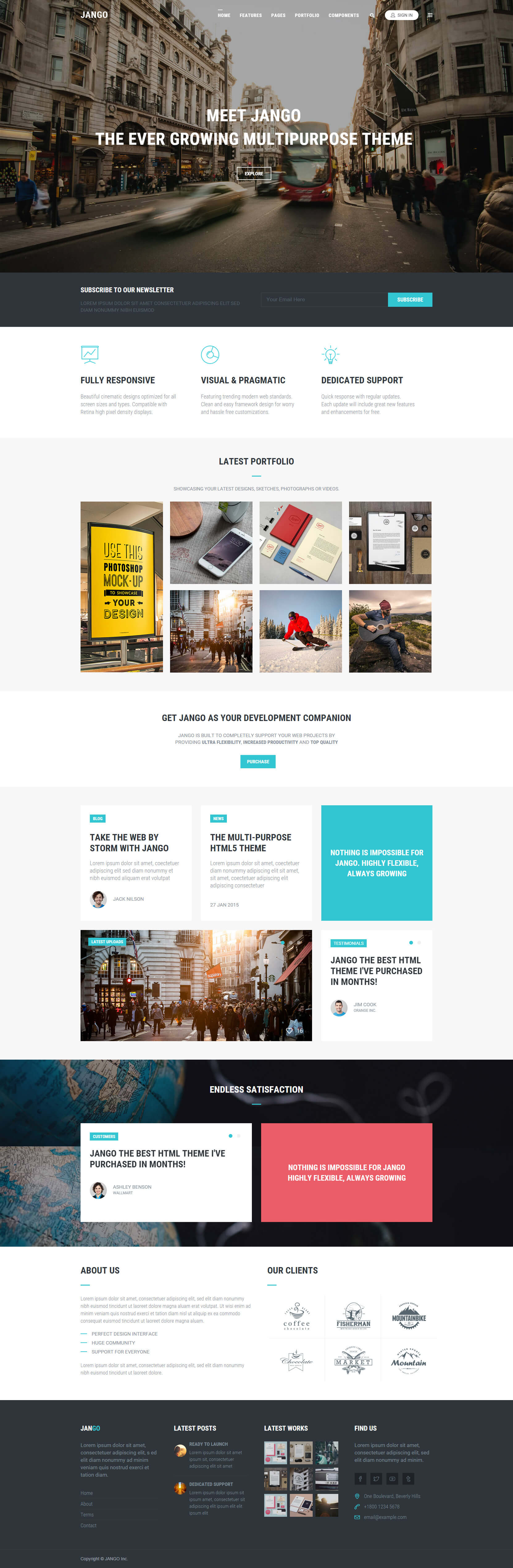In the image, the focus is on an urban city street bustling with traffic and surrounded by towering buildings. At the top of the image, a message reads: "Meet Django, the ever-growing multi-purpose tool." The text is superimposed over the busy street scene. Beneath this main image, there's a smaller section filled with intricate details: 

- There is white text at the very bottom of this section, next to a blue button.
- The top of this lower section also has white text, though it's too small to be easily legible.
- Directly beneath the main image, there's a row of small blue icons accompanied by text that is also difficult to read due to its minuscule size. 

The right-hand side of this lower section contains several components:
- A blue box with blue text at the top.
- A series of small photographs, including an image of a yellow sign that instructs people to wear masks, as well as pictures of telephones, tablets, and various signs.
- There are six smaller photographs grouped together.
- Two horizontal lines are visible, along with another blue button.

Below this, there's a large light blue box featuring a mix of white and blue elements:
- A white area positioned on the left side, intersected by blue elements.
- Additional blue and white sections throughout, including another blue box and a picture marked with a small blue corner in the top left.
- Adjacent to this is another white box with a blue section in the upper left corner featuring a small image.

Following this, there's a darker box displaying images of globes:
- Some of these globe images are accompanied by white boxes with a blue corner in the top left.
- The next section contains another smaller picture.

Towards the end, there's a pink box with white text, accompanied by more white writing above and blue text below. This area is further embellished with various small icons and images, as well as another black section at the very bottom featuring small red details. 

Finally, the image concludes with a display of nine small photographs, aligning with the overall detailed and intricate nature of the entire visual composition.